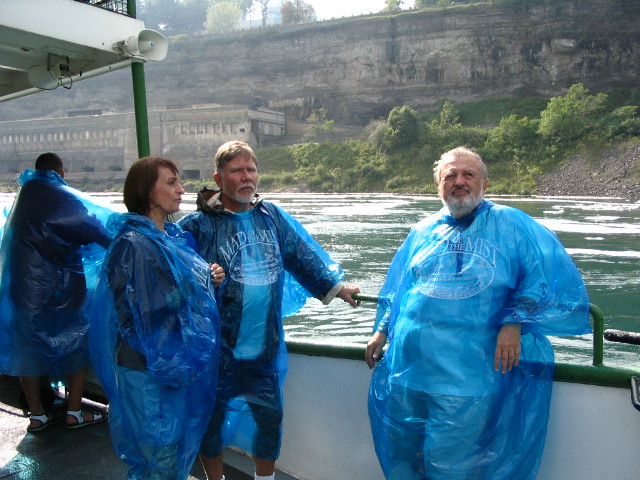In this image, a group of four people is standing on a white tour boat with black railings, likely near Niagara Falls, indicated by the "Maid of the Mist" text on their translucent blue plastic ponchos. The group consists of three men and one woman, all dressed in casual attire including t-shirts, shorts, and capris beneath their rain gear. The man on the far right has distinctive white hair and a beard, while the man next to him sports denim capris and a top under his poncho. The lone woman in the group, who has red hair, can be seen wearing denim shorts or a skirt and a long-sleeve top. Another man, positioned to the left and looking off into the distance, is wearing flip-flops. The boat is positioned near a waterfall or rushing water, with visible trees and an old, dark gray building atop a hill in the background. The water around them is a mix of blue and green, indicating the natural beauty of the location.